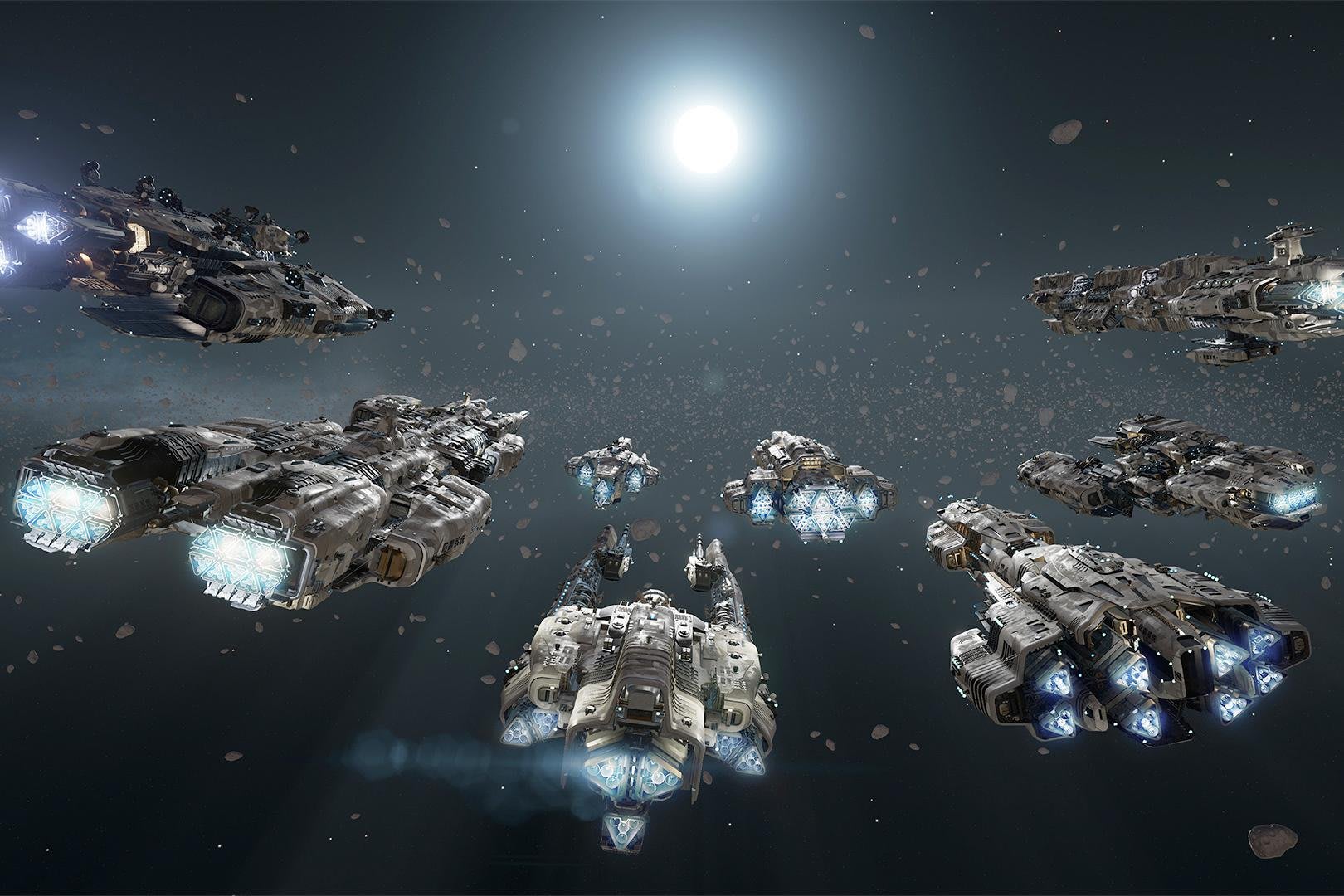The image is a computer-generated depiction with a futuristic setting reminiscent of a space-themed movie or show, such as Star Wars. At the center of the dark, star-filled space is a bright white circular shape, likely representing either a sun or moon, radiating with hues of light blue, turquoise, and dark blue. Surrounding this radiant celestial object are eight large, mechanical-looking starships, characterized by their gray, steel-like panels, and an array of visible guns and compartments. These starships are in a close, orderly formation, with two at the forefront, and the rest spread across the center and right side of the image, their bright blue flames propelling them through an asteroid field filled with brownish-grey rocks. The scene suggests a coordinated movement towards the bright celestial center, giving an impression of a deliberate and possibly strategic maneuver through space.